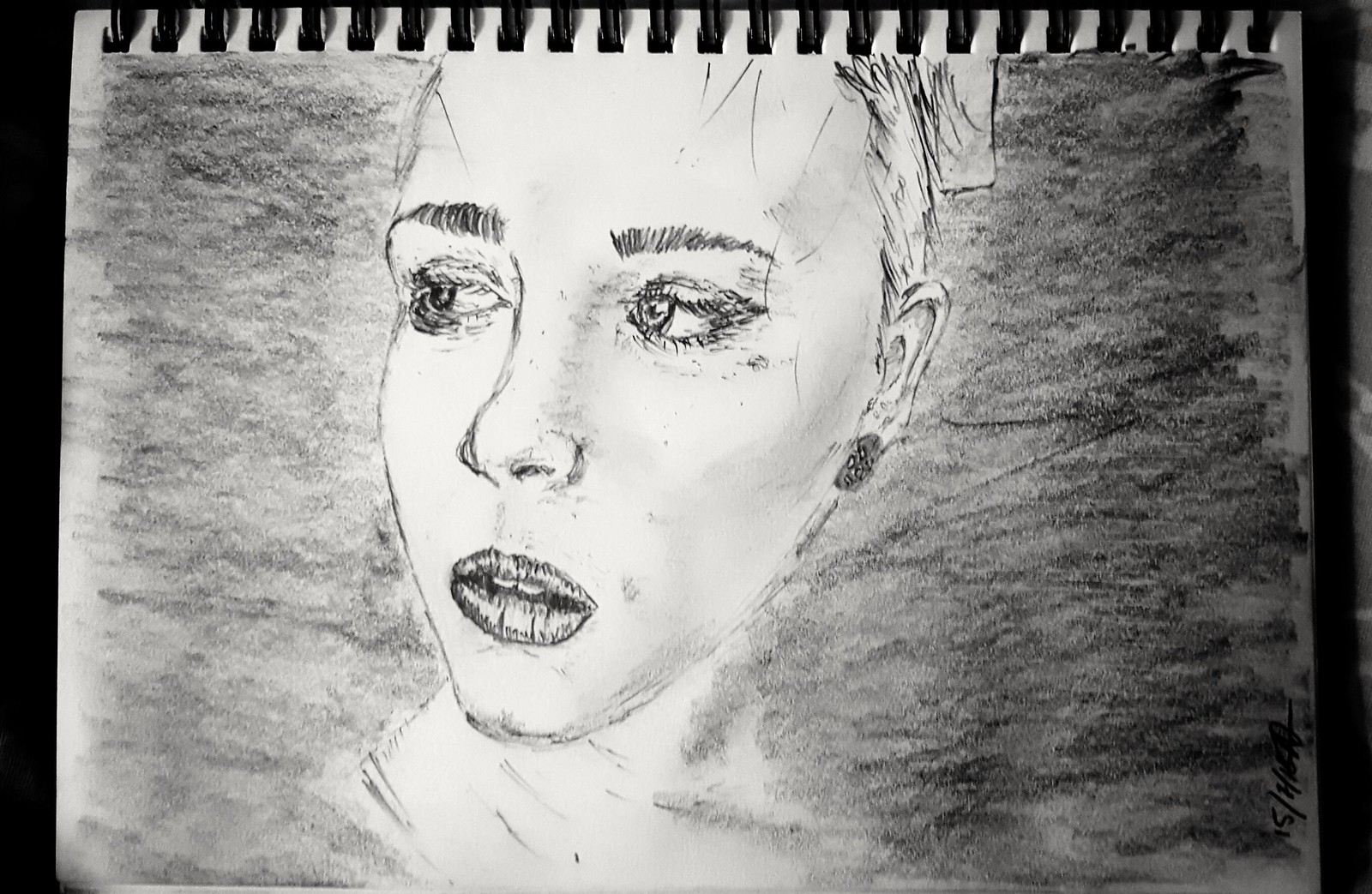This detailed black-and-white sketch is drawn on a sheet of white binder drawing paper, neatly secured within a black-bound sketch pad. The artwork portrays a Caucasian woman adorned with earrings and lipstick, her distinct facial features meticulously rendered. Her expressive eyes are highlighted with defined eyelashes and eyebrows, while delicate strands of hair gracefully cascade over her forehead. The background of the sketch is filled with a subtle, light black shading, providing a gentle contrast to the intricate detailing of her face, including the visibility of two teeth.